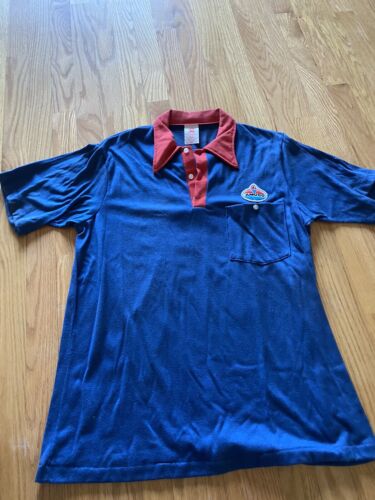The image is a detailed photograph of a blue, short-sleeved polo shirt with distinctive company branding. The shirt features a red collar and a red front placket adorned with two white buttons. Above the left breast pocket, which also has a white button, there is a circular company logo with some writing inside it. The shirt appears freshly unpacked, as indicated by the numerous wrinkles and folds. It is carefully laid out on a wooden surface, likely a floor, with visible wooden boards that transition from a shadowy area at the bottom to a more reflective, brighter area at the top, suggesting natural daylight. The shirt seems to be an extra-large size.